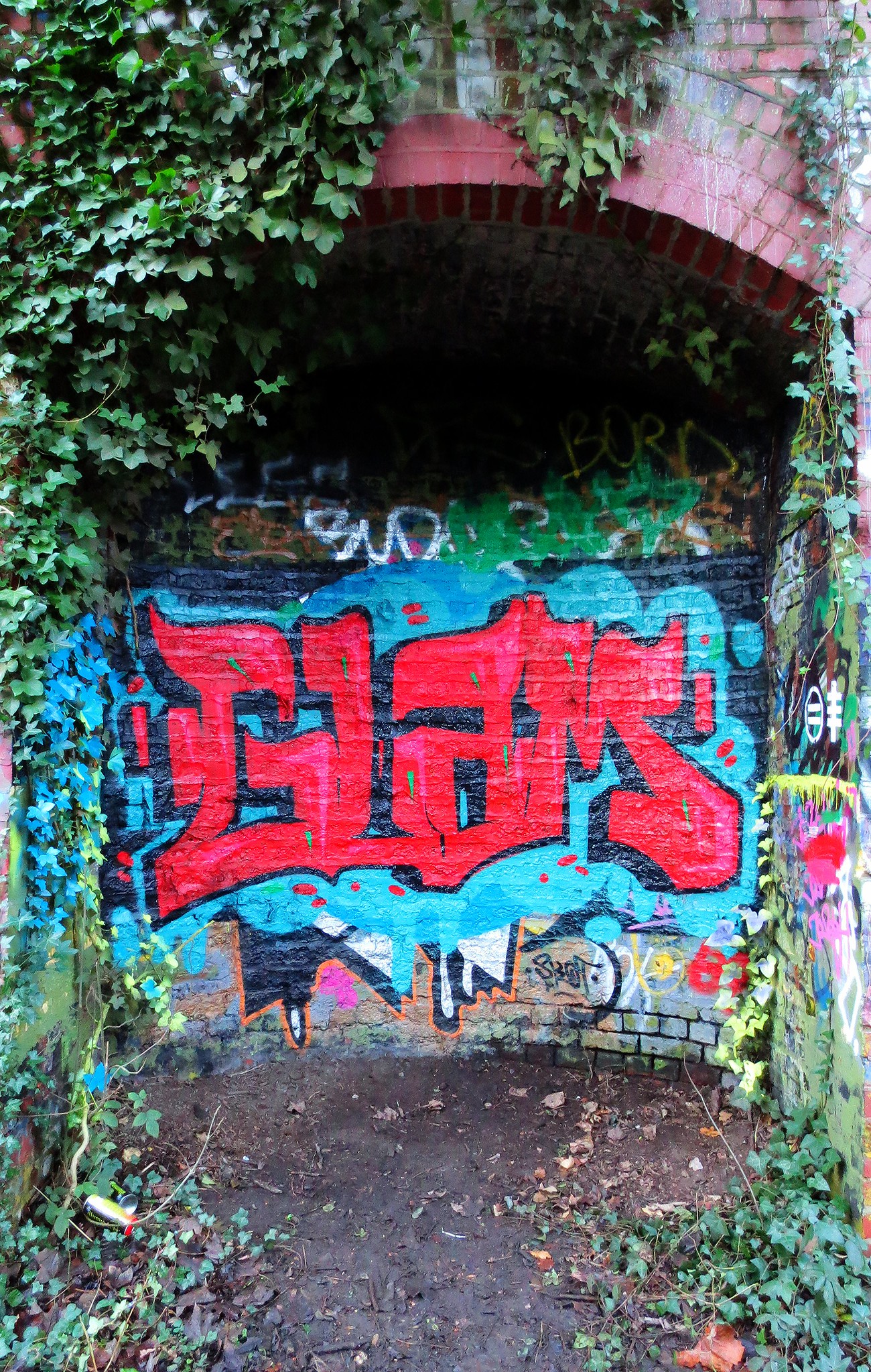The image depicts a garden wall under an obstructed archway. The archway itself is blocked by a brick wall adorned with a variety of graffiti. Central to the graffiti is the word "GLAM" rendered in large, stylized red letters with black outlines, set against a light blue background. This prominent element is surrounded by other graffiti, including words, images, and numbers, both above and below it. Greenery and ivy cascade from the top of the wall, particularly obscuring the upper left-hand corner, and enhance the arch’s structure. On the ground in front of the wall, dirt, additional ivy, and discarded trash, including empty cans, add to the scene's urban decay.